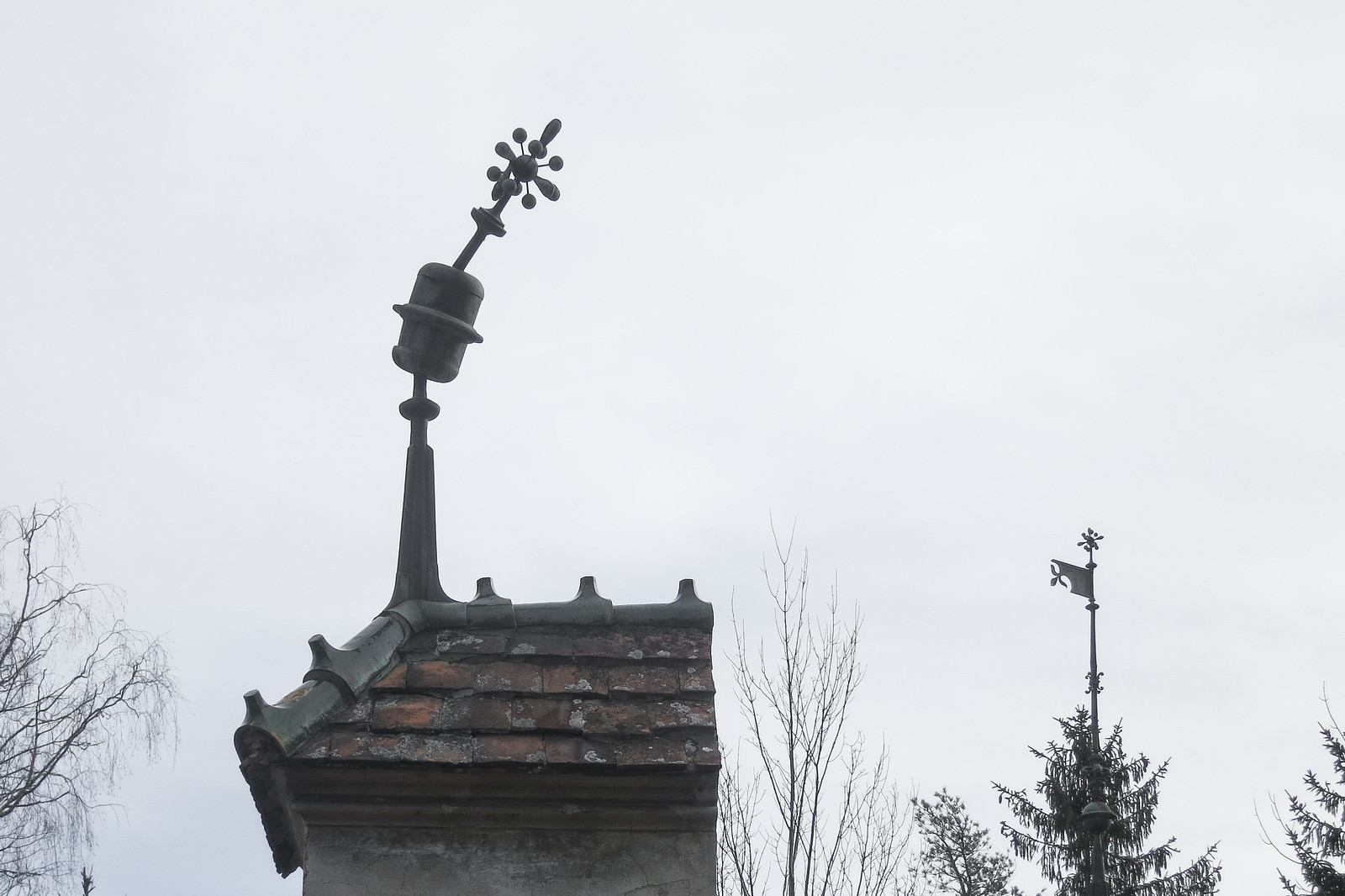The image features a detailed view of what appears to be half of a roof against a gloomy, overcast sky. The upper portion of the image showcases a light blue expanse with heavy cloud cover. Encroaching from the left side are bare tree branches, devoid of leaves. Moving right, the roof is visible with its dirty, shingled surface and gray walls peeking out from the bottom. The roof's trim includes small, smokestack-like protrusions: three along the top and two down the side. At the corner of the roof is a distinctive feature resembling a microphone, tapering up with a central ring and a rod topped with numerous small spheres.

In the distance to the right of this structure, another leafless tree can be seen, alongside a tree with foliage and a large metal object resembling a flagpole. On the rightmost edge, partially obscured by branches, is what seems to be a trunk with leaves. The overall scene hints at an incomplete structure set within a wooded area, punctuated by several mysterious metal installations that might be communication or weather monitoring equipment.